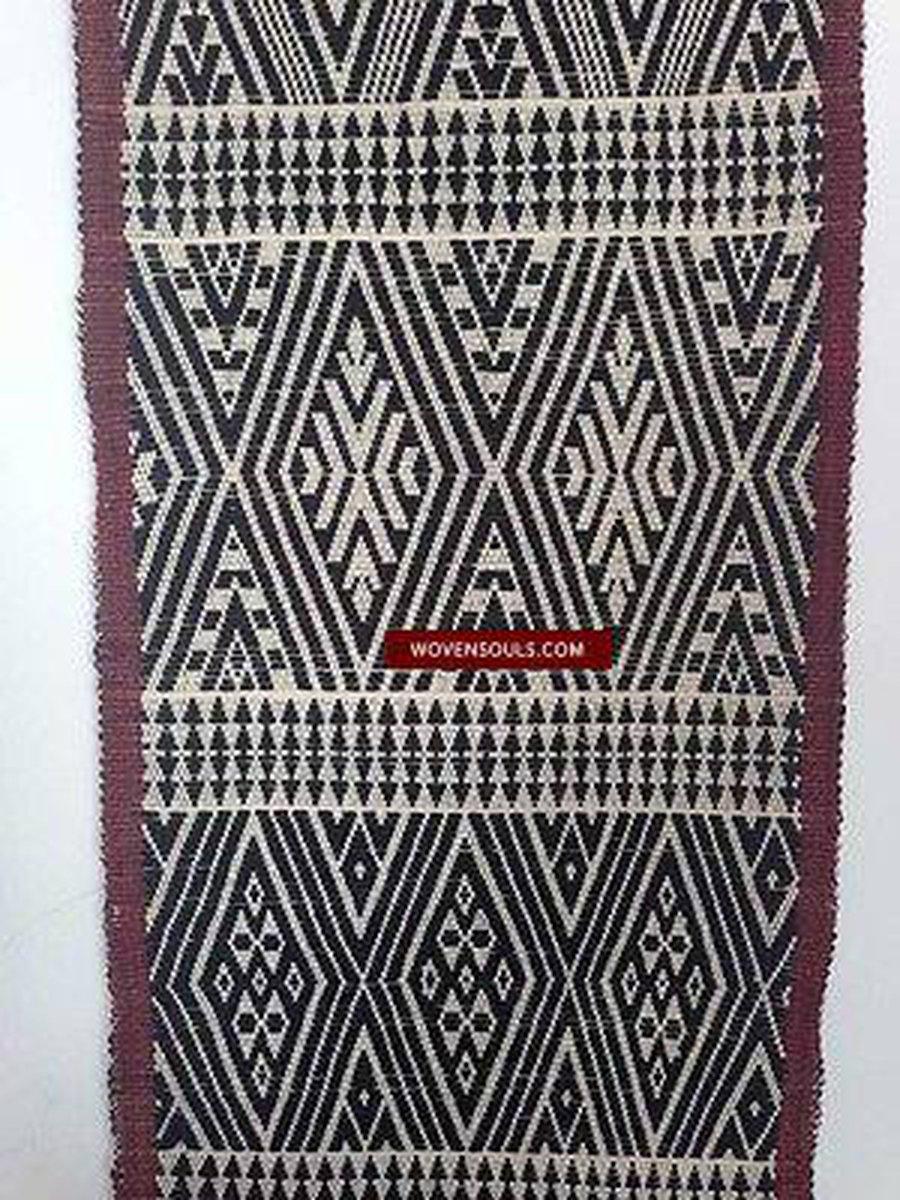This is a detailed photograph of a woven wall hanging, possibly a rug, predominantly in black and white. The centerpiece of this textile art features the text "wovensouls.com" in red. The overall pattern consists of large diamond shapes that contain intricate, repeating designs such as diamonds within diamonds and chevron patterns. The diamonds' interiors alternate between black backgrounds with white designs and simple black and white contrasts. The piece is bordered with a subdued eggplant or mauve purple trim and is set against a white background. The tapestry also displays rows of small triangles, with two of the triangles in each row facing upwards and the other two facing downwards. This arrangement of triangles occurs in rows across the tapestry, interspersed between the larger diamond patterns. The combination of these geometric shapes and colors lends the piece a Native American aesthetic, enhanced by its detailed craftsmanship and symbolic motifs.